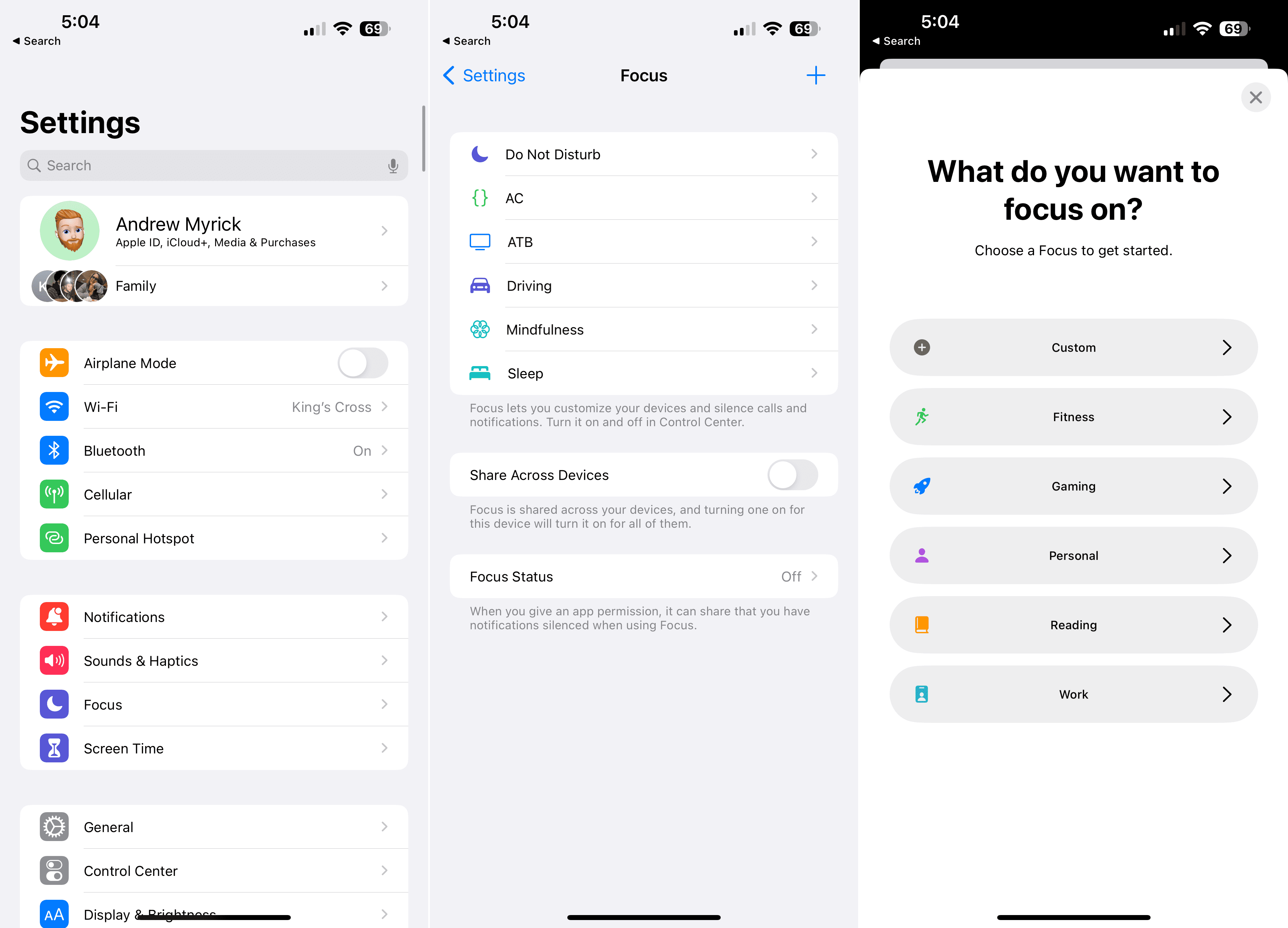This image displays three distinct settings pages on cell phone screens, each with a light gray background.

The first screen, on the left, features a timestamp at the top left displaying "5:04." Below it, there is a label "Switch," followed by the bold black text "Settings." Underneath the settings header, there is a search bar. Below the search bar appears an avatar of a Caucasian male with red hair, a red beard, and blue eyes, labeled "Andrew Myrick." The screen further indicates options related to Apple ID, iCloud, and media and purchases. Beneath this section, icons for various settings appear in sequence, including "Family," "Airplane Mode," "Wi-Fi," "Bluetooth," "Cellular," "Personal Hotspot," "Notifications," "Sounds & Haptics," "Focus," "Screen Time," "General," "Control Center," and "Display."

The middle screen also shows "5:04" as the timestamp, beneath which the header "Settings" is visible. This page focuses on the "Do Not Disturb" settings, listing various modes such as "Do Not Disturb," "AC," "ATB," "Driving," "Mindfulness," and "Sleep." The "Share Across Devices" option is visibly toggled off, followed by a similarly off "Focus Status." The page prompts "What do you want to focus on?" and underneath, it suggests "Choose a focus to get started" with options like "Custom," "Fitness," "Gaming," "Personal," "Reading," and "Work."

The detailed layout and clear organization of each screen's settings facilitate user navigation and personalized configuration.